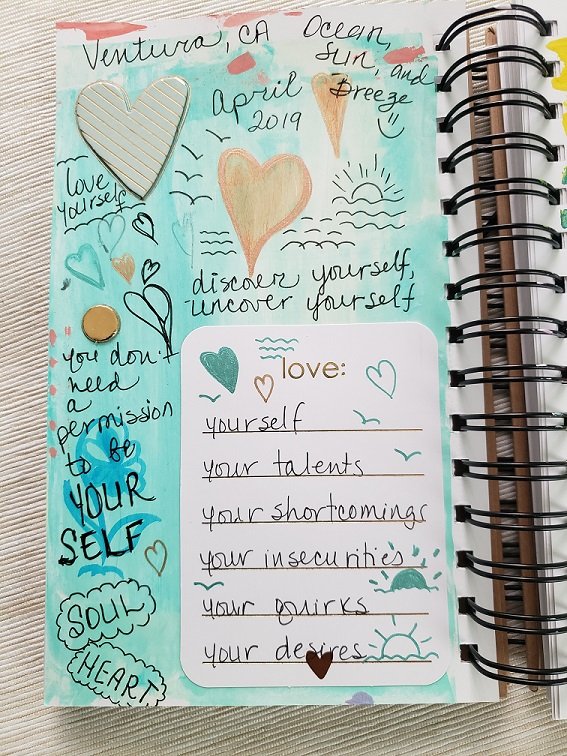This image depicts a page from a spiral-bound journal designed specifically for journaling, featuring elaborate pre-printed graphics and text prompts. The page is adorned with a turquoise-green background that evokes an oceanic theme, including illustrations of waves, a rising sun, and seagulls. Hand-drawn and printed hearts in various shades of orange and blue are scattered across the page. Prominent phrases such as "Love yourself," "Discover yourself," "Uncover yourself," and "You don't need permission to be yourself" are seamlessly integrated into the design, along with the words "soul" and "heart" inscribed within cloud shapes.

Personal annotations by the journal owner add a sentimental layer to the page, including the location "Ventura, California," the words "ocean, sun, and breeze" marked with a smiley face, and the date "April 2019." At the top of the page, beneath the heading "love," the individual has listed self-reflective terms: "yourself, your talents, your shortcomings, your insecurities, your quirks, and your desires." Overall, the page serves as a colorful, motivational canvas blending pre-formatted prompts with personal expression.